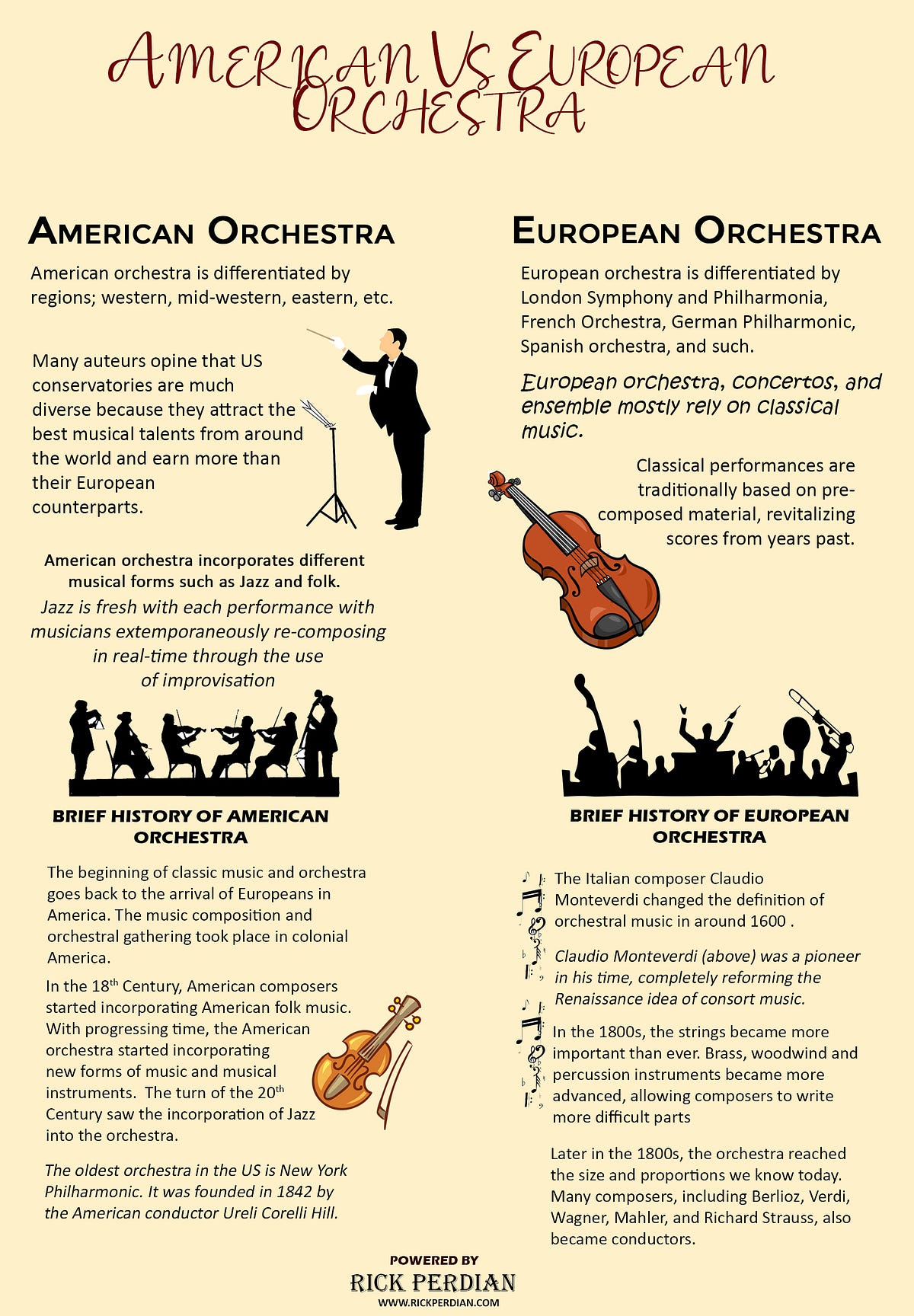This image is a detailed informational flyer or webpage titled in a classic script font: "American vs. European Orchestra." It is divided into two primary columns. On the left side, under the header "American Orchestra," there is a section titled "Brief History of the American Orchestra" with information discussing how American orchestras, defined by regions such as western, midwestern, and eastern, attract diverse musical talents from around the world and tend to earn more than their European counterparts. This section is illustrated with a picture of a conductor leading the orchestra. It highlights the incorporation of various musical forms like jazz and folk, noting jazz's unique quality of live improvisation.

On the right side, under the header "European Orchestra," the section titled "Brief History of the European Orchestra" provides details on the distinctions between various European orchestras, such as the London Symphony, Philharmonia, French Orchestra, German Philharmonic, and Spanish Orchestra. This column includes a picture of a violin and elaborates on how European orchestras predominantly focus on classical music, performing compositions that revitalize historical scores. The layout features black and white silhouette drawings representing small orchestra ensembles on both sides.

At the very bottom of the page, it states "Powered by Rick Perdean," with a URL (www.rickperdean.com), suggesting that this detailed comparative information is sourced from his website.